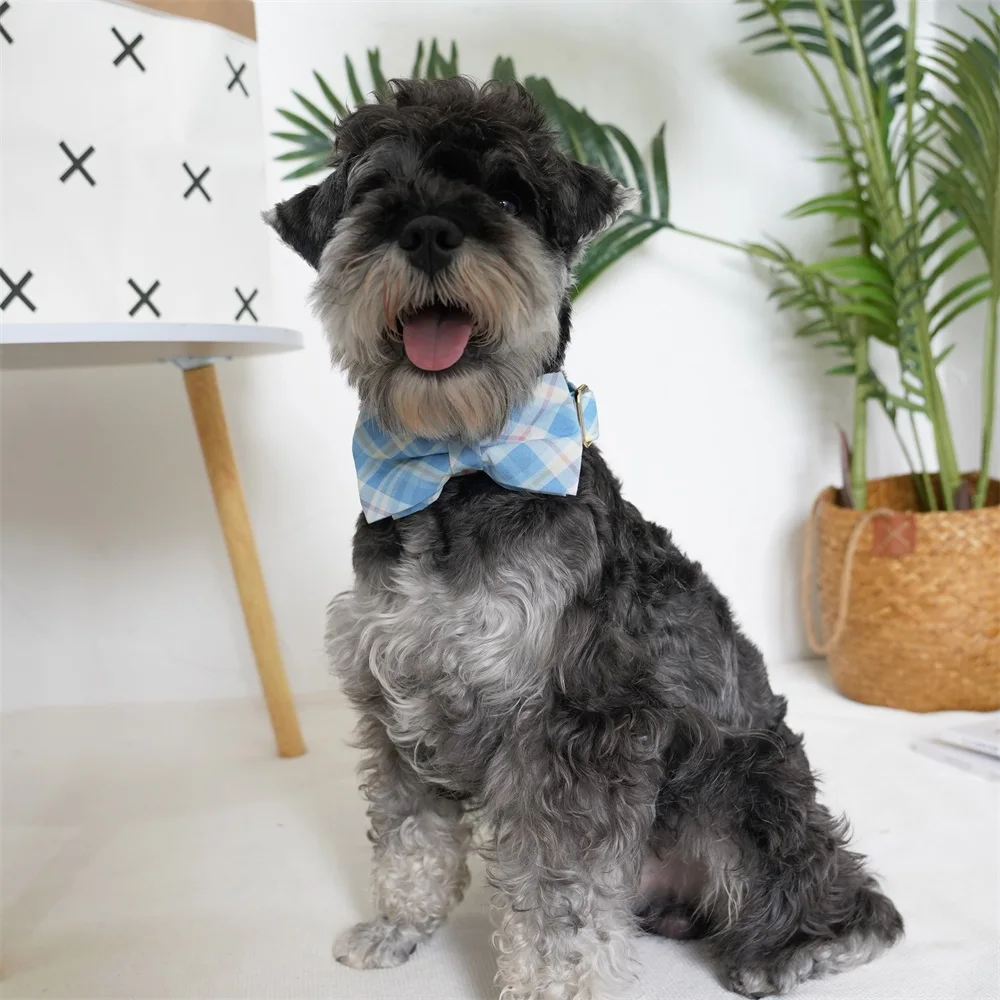In this detailed portrait we see a small schnauzer with a short, puppy cut sitting upright on a light gray, nearly white, floor in what appears to be a living room. The dog's fur is a mix of black and gray, with some light yellow around its mouth, and it has a distinctive black mask over its eyes. The schnauzer is looking directly at the camera with its mouth open and tongue visible. Adorning its neck is a charming blue and white plaid bow tie. To the right of the schnauzer, there is a green house plant in a light brown wicker basket. To the left of the dog, there is an object that looks like a white piece of paper with black X's held up by a light brown stand. The background features a light gray wall with a reflection of white light, enhancing the overall bright and cheerful ambiance of the scene.